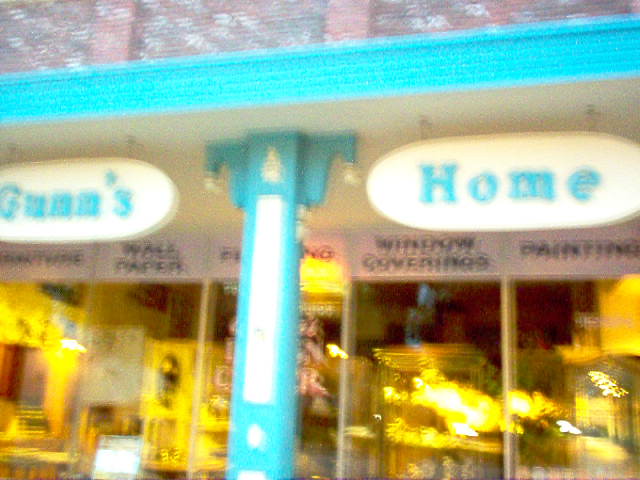The photograph captures the exterior of a storefront, featuring a primarily brick building with a red and white, slightly brownish hue at the top. Below the brickwork, there's a vivid, sky-blue awning extending across the front, highlighted by a matching blue column with a white rectangular section in the center and a touch of gold design at the top. The image appears overexposed and somewhat blurry, making intricate details challenging to discern. Hanging above the storefront are two tan, oval-shaped signs with blue lettering: the left sign reads "Gunn's" and the right sign says "Home." Large glass windows front the store, revealing an illuminated interior that suggests it is a furniture store, displaying items like desks, lamps, and various furnishings. Visible signage above the windows lists offerings such as wallpaper, furniture, window coverings, and paintings. The store's ambiance is a blend of yellow, gold, and brown tones, creating a warm and inviting display.